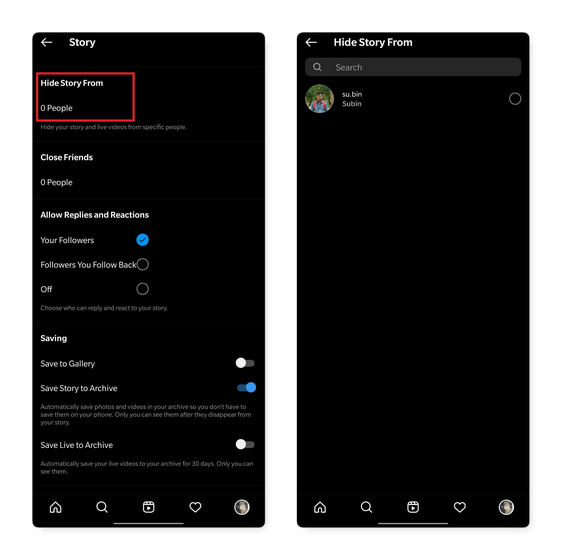The image is a side-by-side comparison of two screenshots taken from what appears to be an Instagram settings page on a mobile device. Both images feature a predominantly black interface with identical bottom navigation bars consisting of five icons: a house, magnifying glass, play button, heart, and a profile picture from left to right.

**Left Image:**

The left screenshot focuses on various privacy and save settings for Instagram stories:
- The phrase "Hide Story From 0 People" is highlighted in a red square box, indicating the option to hide stories and live videos from specific users.
- Under this, the "Close Friends" list currently includes 0 people.
- For allowing replies and reactions, options available are "Your Followers," "Followers You Follow Back," and "Off."
- In the "Saving" category:
  - "Save to Gallery" toggle is turned off.
  - "Save Story to Archive" toggle is turned on with the description explaining that photos and videos are automatically saved to your archive and visible only to you after they disappear from your story.
  - "Save Live to Archive" is toggled off, with a note stating live videos can be automatically saved to your archive for 30 days and are visible only to you.

**Right Image:**

The right screenshot appears to show an example of hiding stories from specific users:
- The same "Hide Story From" option now displays a user profile, though difficult to discern, with the username or name partly visible as "Subin twice."

This comparison illustrates the steps and options available in Instagram for customizing who can view your stories and how you can manage the storage of your story contents.